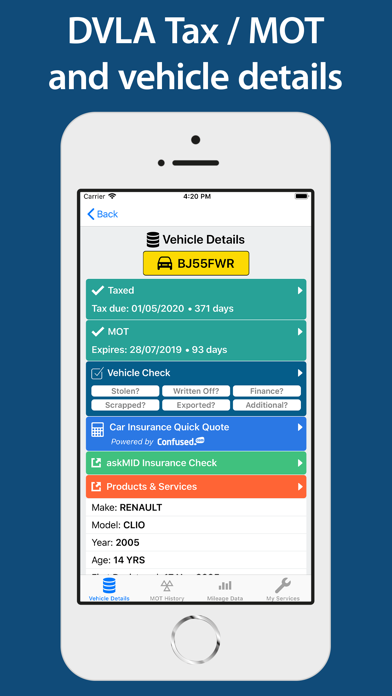The image features an interface layout, which prominently displays blue rectangles forming the background at the top. In white text, it reads "DVLA Tax / MOT and Vehicle Details." Below, a smartphone is depicted in light gray with a black camera dot at the top and another sensor dot with an adjacent dash next to it. The phone screen contains a black outlined rectangle displaying various elements.

At the top left of the screen, there's an arrow pointing left labeled "Back," situated near an icon resembling a drum under the heading "Vehicle Details." A yellow rectangle features a car icon and the text "BJ55FWR." Adjacent to this is a blue-green rectangle with a check mark, accompanying some text and a right-pointing arrow. Another greenish box, also with a check mark, follows the same pattern with text and a right-pointing arrow. Additionally, a blue box has a check mark within a square, text, and a right-pointing arrow.

Below these elements, there are six white buttons arranged in two rows of three, each containing text. A blue rectangle underneath them includes an image resembling a calculator, text, and a right-pointing arrow. Further down, a green box is shown with an undistinguishable image, accompanied by text and a right-pointing arrow. An orange rectangle follows, featuring the same logo but with an orange background, having another right-pointing arrow and some text.

Towards the bottom, there is a blue barrel-like icon with text beneath it. Below this are three triangles touching at their top points with text below, followed by another section with lines and further text. An icon resembling a tool with accompanying text is also present. The layout concludes with a silver circle situated at the very bottom of the screen.